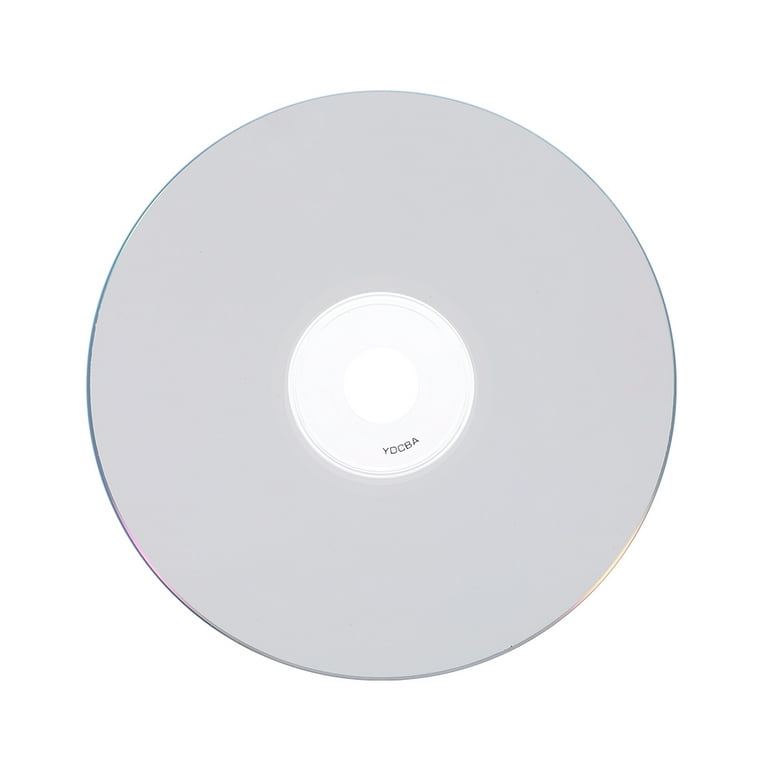The image shows a close-up photograph of the underside of a CD. The CD is positioned flat on a completely white background, emphasizing its circular shape. The outer rim of the CD features a multicolored, prism-like border that contrasts with the predominantly light bluish-gray surface of the disc. In the center of the CD is a small, clear region with finer detailing, including small black capital letters that read "Y-D-C-B-A." The CD also has a central hole typical of such discs. Despite the lack of visible grooves or lines on the surface, the characteristic reflective rainbow edge unmistakably identifies it as the back of a CD.